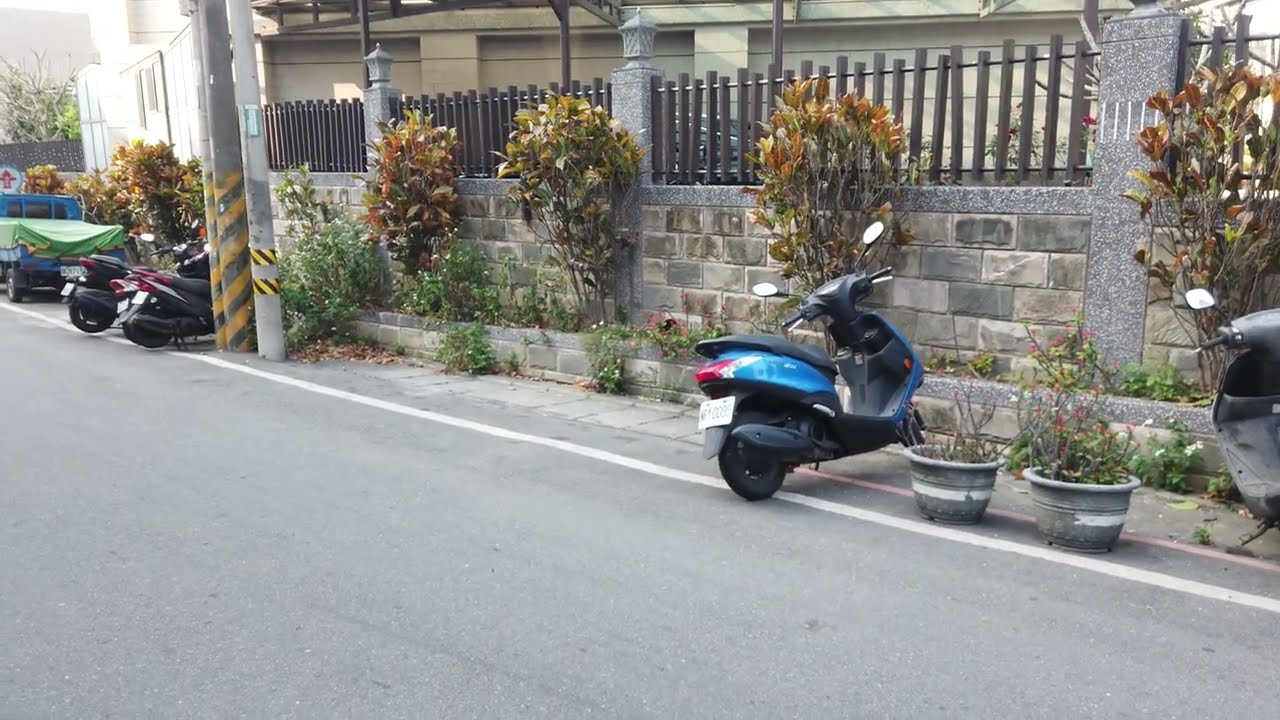In the image, there's a blue scooter with a black seat parked on the side of a road. To its right are two concrete flower pots—one white and one red—positioned between two painted lines on the road. The scooter is parked in front of a building made of gray bricks, with a black fence gate atop the brick wall. Concrete posts stand between sections of the fence, each topped with a lantern-style light. Sparse greenery, including bushes and small trees, is present around the building. There are no people in the scene, suggesting it is either early morning or afternoon given the bright lighting. To the right of the blue scooter, another scooter is partially visible. To the far left, there are two additional scooters, one red and the other dark-colored, along with a partial view of a blue pickup truck carrying something covered by a green tarp. The overall scene suggests an urban or residential area, likely in an Asian country due to the construction style.